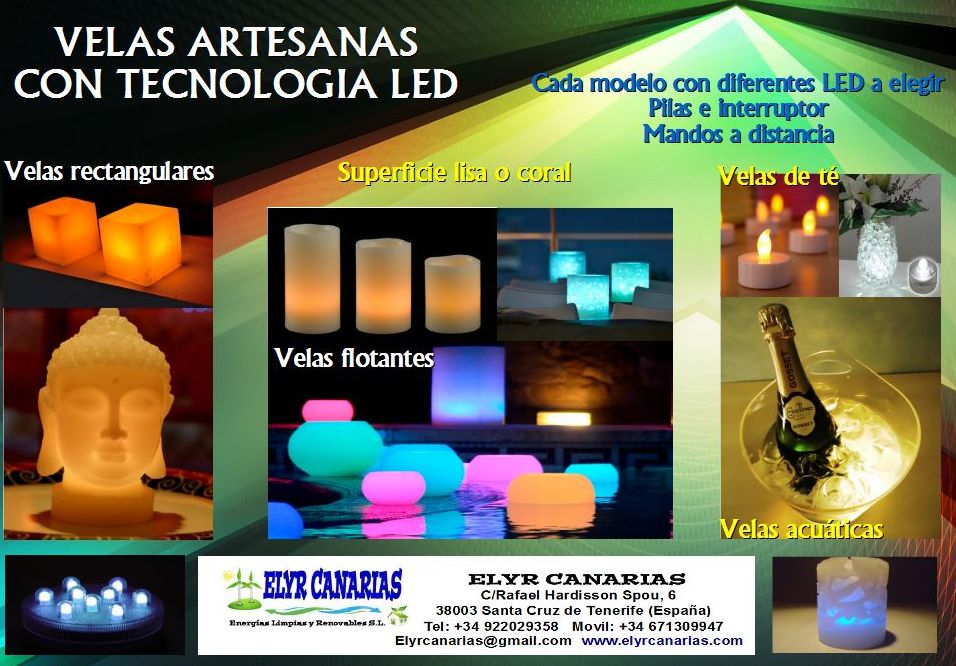This detailed horizontal rectangular advertisement features a green structure at the center and right, resembling a building with various openings showcasing LED products for sale. The top right of the image prominently displays the text "Velas Artesanas con Tecnología LED" in white Spanish letters, with additional smaller white text below. 

In greater detail, the advertisement is divided into three primary sections:

1. The left section titled "Velas Rectangulares" features rectangular LED lights, some resembling faces, categorized as Buddha LED lights.
2. The central section highlights "Velas Flotantes," showcasing standard large candles referred to as floating candles with smooth or coral surfaces. Also depicted are tea lights (Velas de Te) and vases illuminated from inside.
3. The right section describes aquatic-themed lights, including those that can be placed in water (Velas Acuáticas) and a champagne bottle illuminated from beneath.

The bottom section contains a white label with black text on the right, likely showing the company's contact information: Elir Canarias, located in Santa Cruz de Tenerife, Spain. To the left of the label is a blue logo.

The background transitions through a spectrum of colors from orange to green, adding visual appeal to the advertisement that aims to guide potential customers to their store in Spain.